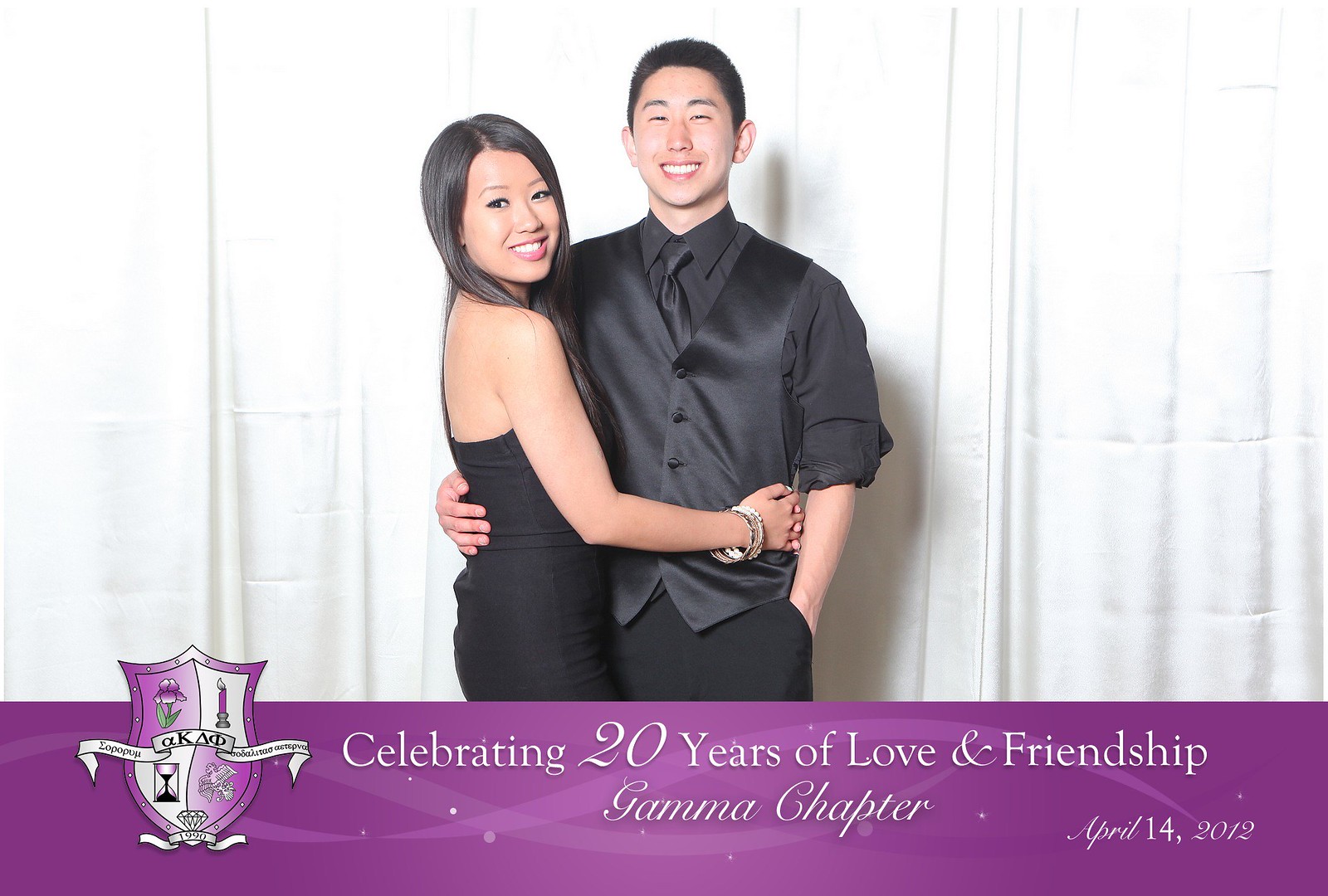This is a horizontally aligned rectangular picture featuring a happy couple standing in front of a tall white curtain. The man, standing on the right, is a young Asian man dressed in a black vest over a black dress shirt with a black tie and black slacks. His sleeves are rolled up, and he has short black hair. He has his arm around the woman's lower back. The woman, standing to his left, has long black hair and is smiling brightly. She is wearing a tight-fitting sleeveless black sheath dress and some bracelets, and she has both of her hands around his waist. At the bottom of the picture is a purple rectangular section with white print that reads, “Celebrating 20 Years of Love and Friendship, Gamma Chapter,” and to the lower right corner, “April 14th, 2012.” There is also a symbol—a crest with various emblems—next to the text.